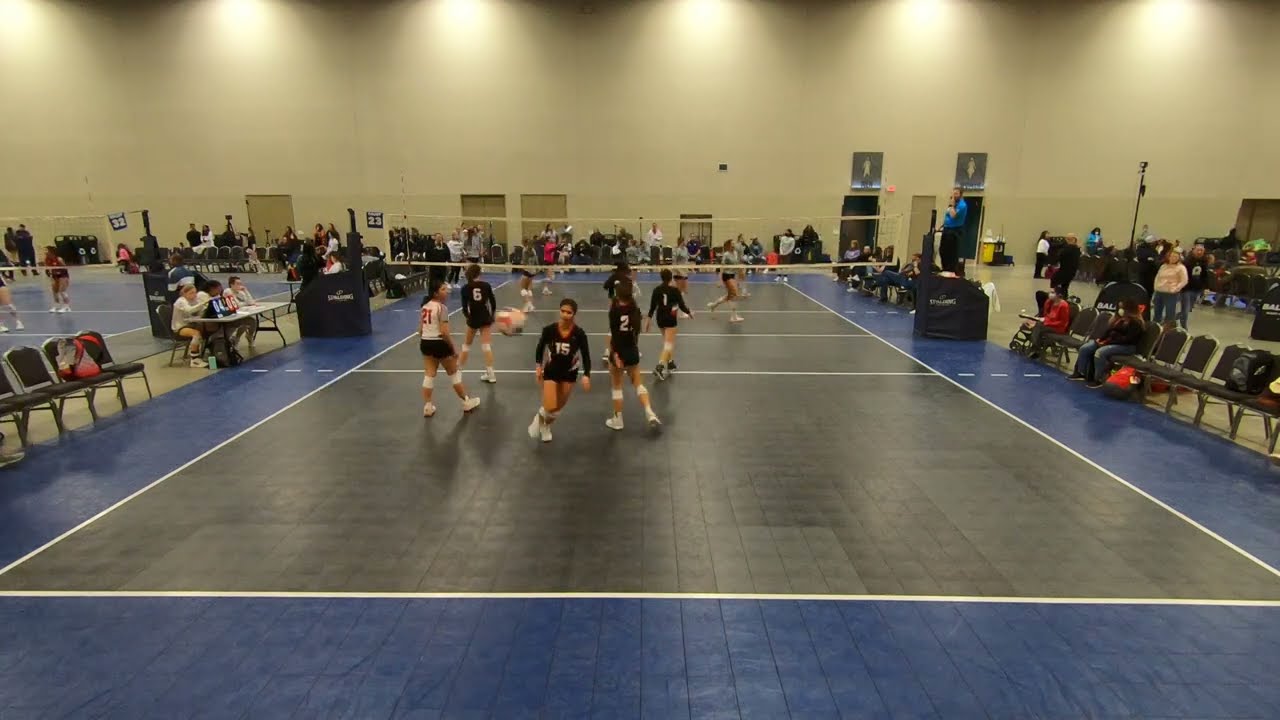The photograph captures an energetic scene inside a sprawling gymnasium, focused primarily on an active women's volleyball match. The game unfolds on a gray volleyball court, framed by dark blue borders. Ten players are intensely engaged in play, with some clad in black shorts and white jerseys, while others sport dark tops—each numbered clearly on the front and back. The vantage point is slightly elevated, providing a comprehensive view of the action across and behind the net. 

Spectators, although not forming a substantial crowd, are positioned along the far wall, flanked by gray seating, observing the competition. Additional viewers are dispersed along either side of the court. Two judges, each perched on podiums adjacent to the net, oversee the proceedings. To the left side of the court stands a long table where three officials appear to be keeping score, and there is another volleyball court partially visible to the left, indicating the gymnasium's large capacity. Several doors punctuate the opposite wall, and various cameras and people are visible on the right side of the image, capturing the dynamic atmosphere of the event.